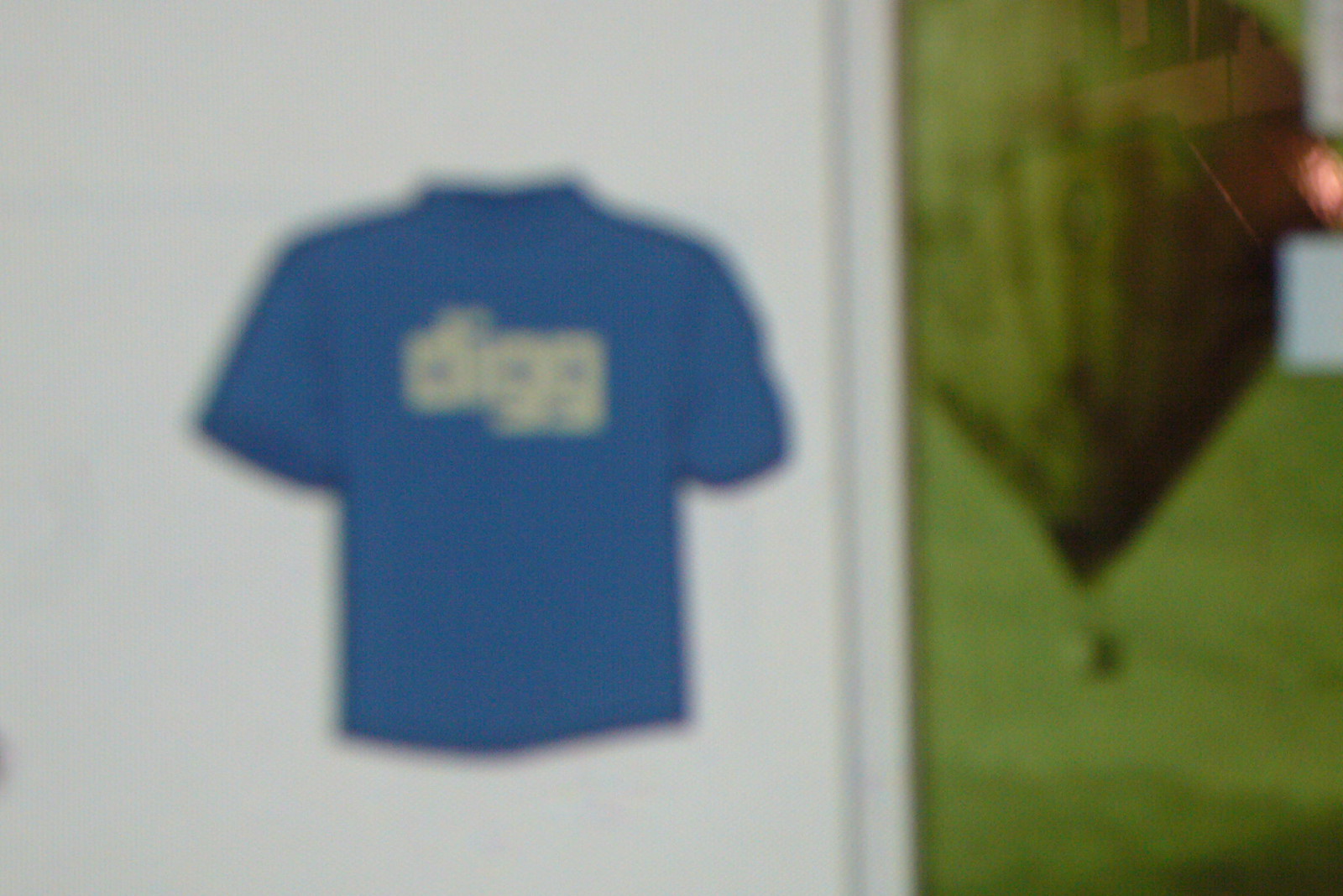This image features a screenshot of a computer monitor displaying a product image of a blue t-shirt. The picture appears somewhat blurry but prominently showcases the blue shirt with the text "DIGG" visible on it, likely indicative of a popular website. To the right side of the image, elements of the computer desktop are visible, including a background featuring a vibrant scene of a hot air balloon floating over a green field. The product image itself is set against a stark white background, emphasizing the blue t-shirt. This detailed view suggests the photo is a blend of a product advertisement and a glimpse of the user's desktop environment.